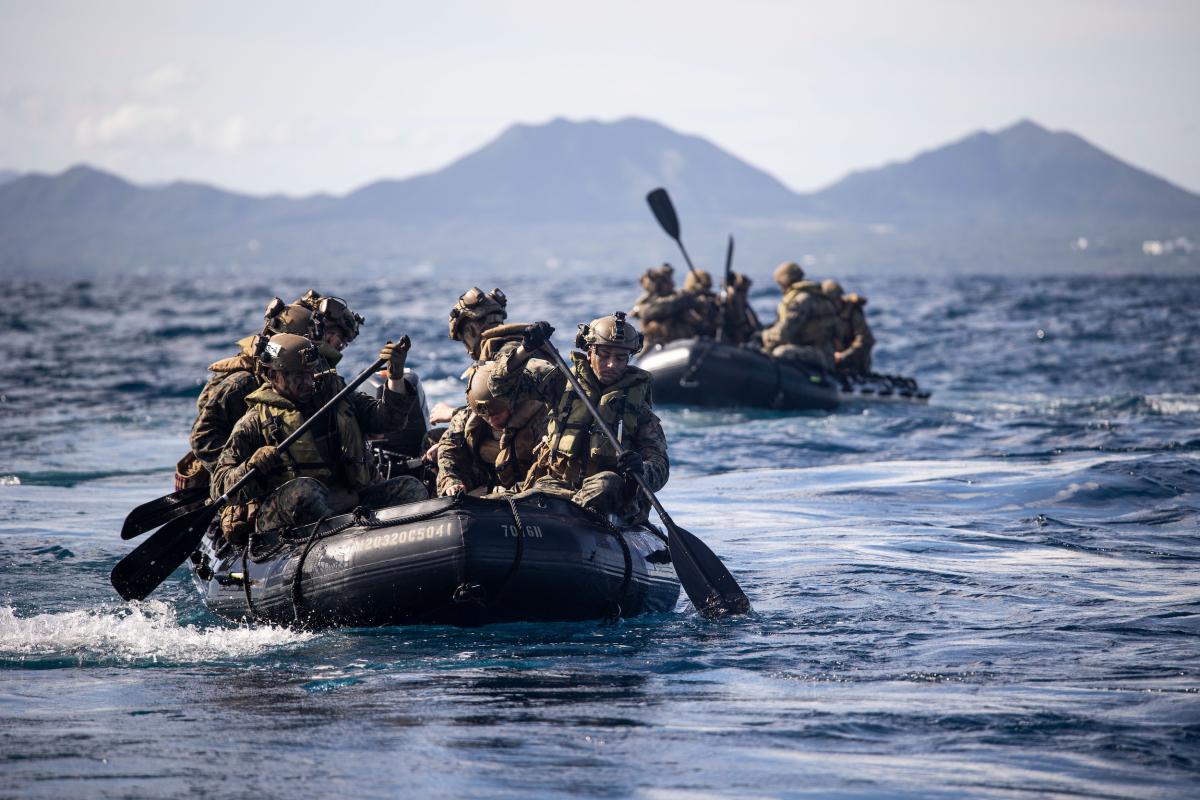This image captures a tense and dynamic scene of military personnel, possibly Navy SEALs, navigating two black rafts on a choppy, dark blue ocean. The soldiers, whose precise branches are not distinctly identifiable, are clad in green-brown uniforms and helmets. Each raft is manned by five to seven individuals, all vigorously using black oars to propel the boats forward, indicating a probable training exercise. While a motor is visible on the leading raft, its presence on the second, partially obscured raft, remains uncertain. The backdrop features muted, imposing mountains, adding to the rugged and intense atmosphere of the image. Their collective effort against the tumultuous waves highlights their dedication and coordination in this seemingly strategic maneuver.